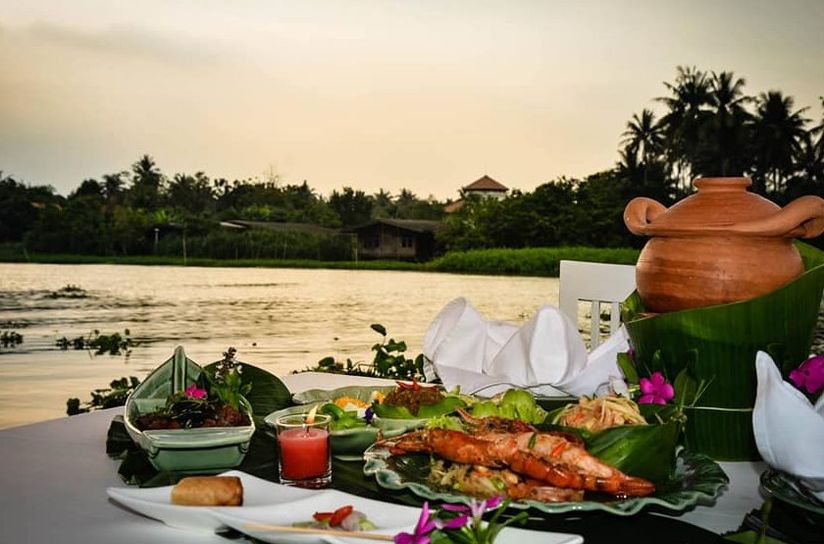The image captures an outdoor dining scene situated by the water under an overcast sky, giving a serene ambiance just before nightfall. In the foreground, a grey table holds an array of dishes with a variety of foods. A prominent green ceramic boat-shaped platter features in the left corner, while a white ceramic three-part plate beside it contains what appears to be an egg roll, vegetables, and purple flowers. Adjacent is a white vase, and a glass jar with a red candle casts a warm glow. The table also hosts a white bowl and a large green container holding a brown basket, adding to the eclectic setup. The meal likely includes dishes like lobster tail and sushi, presented on green and white plates. Behind this setup, the scene transitions into a peaceful waterscape dotted with lily pads and bordered by lush green space. A house and a tower are visible in the background, contributing to the picturesque setting. The presence of trees and the lack of boats further enhance the tranquil atmosphere.